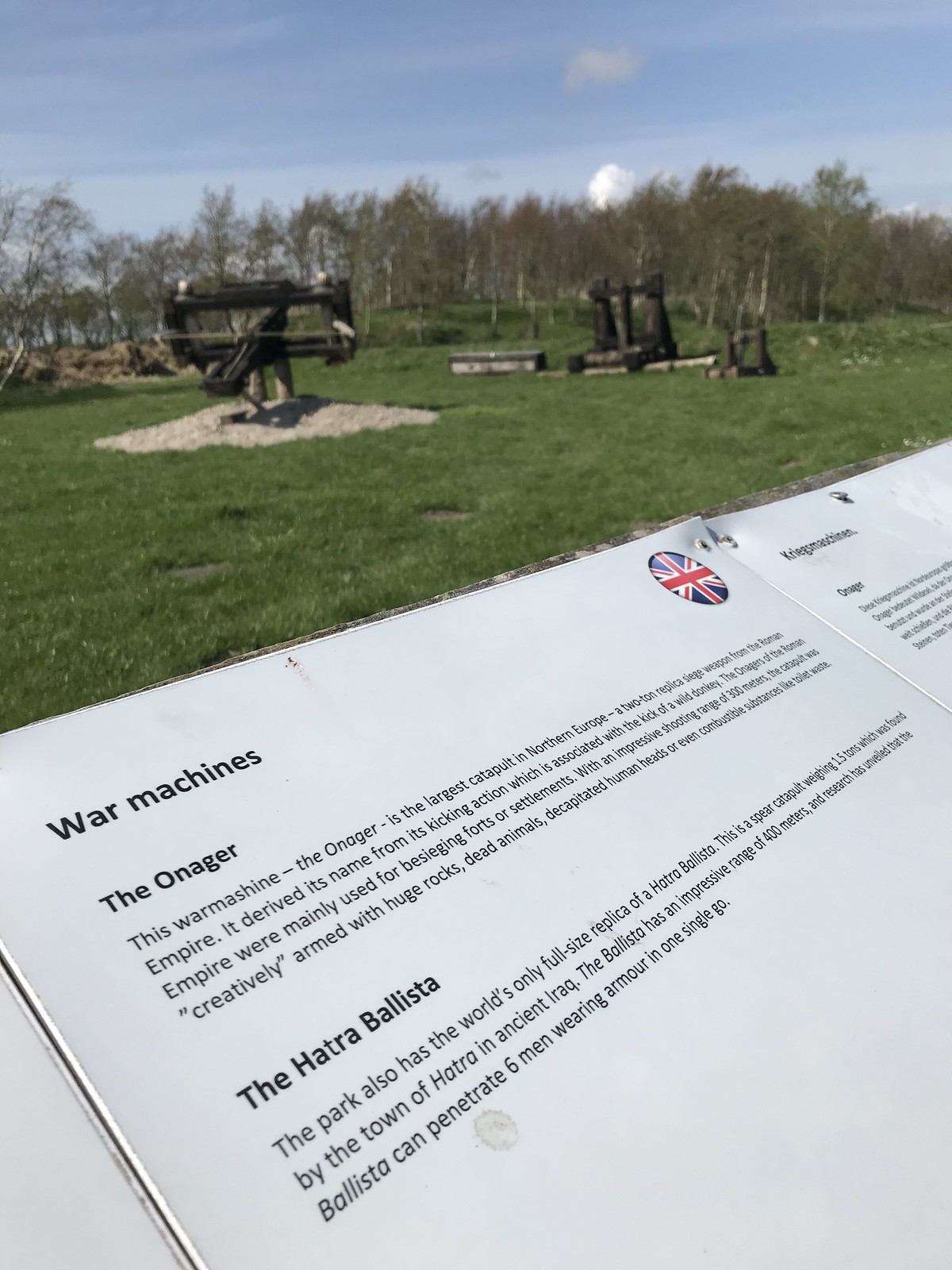The photograph captures a historical war memorial situated in a park, featuring two prominent ancient war machines displayed on a grassy field with a backdrop of trees and a clear sky. In the foreground, a white sign with black lettering and a British flag symbol informs visitors about these preserved relics. One machine, named the Onager, is a two-ton catapult that derives its name from the kicking action of a wild donkey, hailing from the Roman Empire and noted as the largest catapult in northern Europe. The second machine, the Hatra Ballista, is a 1.5-ton spear catapult, historically found in the ancient town of Hatra in Iran. Constructed from wood and metal, these war machines appear small from a distance but are substantial in size. The plaque offers bilingual information, predominantly in English with some content in German, enhancing the educational experience of this outdoor display. The entire scene is devoid of people, emphasizing the solemn, contemplative nature of the memorial.